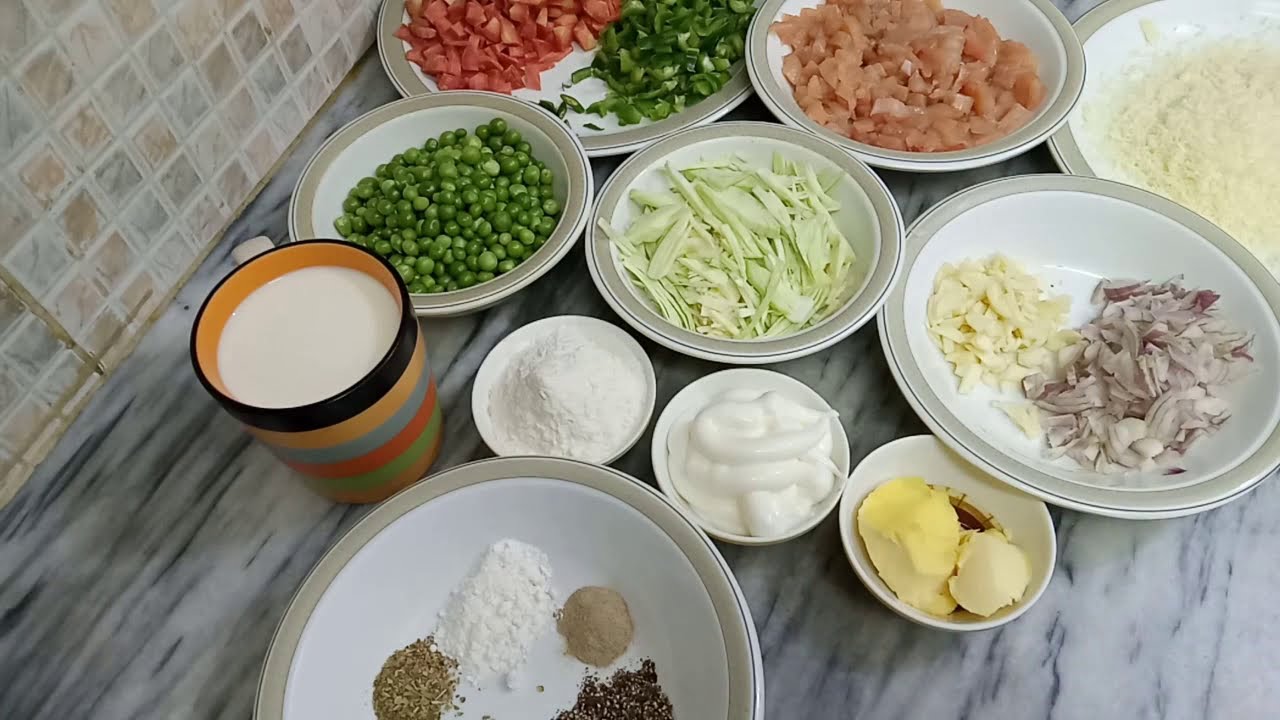On a gray and white mottled marble countertop with a light brown tile backsplash, a neatly arranged array of white dishes and ramekins are filled with various ingredients, suggesting meal preparation. At the forefront, there's a round plate with small piles of different spices, hinting at salt, pepper, and other seasonings. Nearby, three small bowls contain flour, a thick white substance possibly sour cream, and a yellow one that might be butter. A multicolored coffee mug filled with milk sits next to these bowls.

Further back, bowls contain meticulously prepared ingredients: green peas, shredded lettuce, chopped purple onions mixed with another vegetable, chopped raw chicken, and a mixture of green and red bell peppers. A larger bowl holds different little piles of herbs. The overall scene suggests a detailed and well-organized setting for preparing a complex dish, possibly a taco or fajita meal.